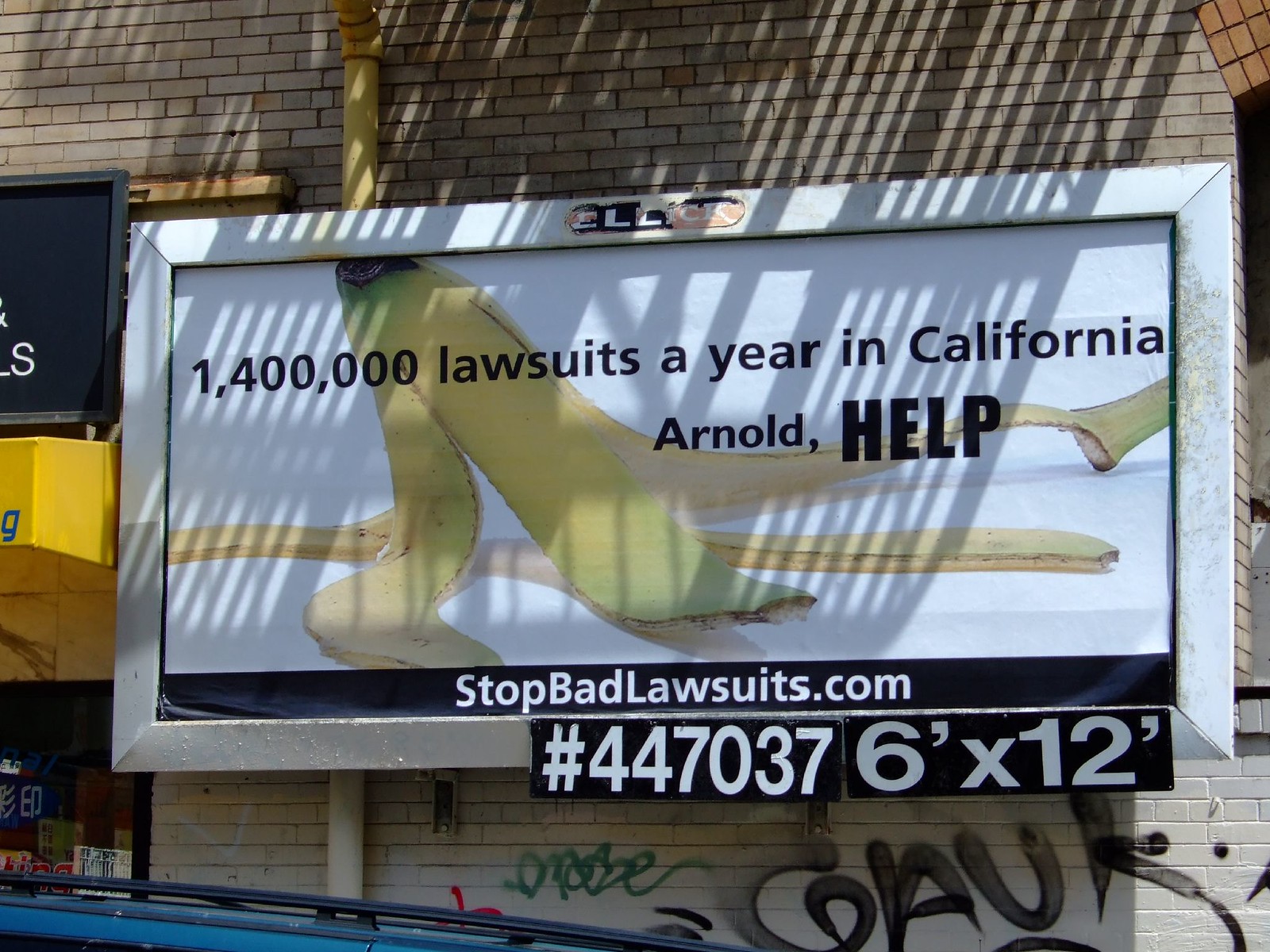The image depicts a large silver-framed billboard mounted on a light gray brick building with noticeable graffiti and black lettering below it. The billboard, approximately six feet by twelve feet in size, prominently features a splayed-out banana peel on a white background. Above the banana peel, bold black text states, "1,400,000 lawsuits a year in California. Arnold, HELP." The word "HELP" is emphasized in all caps and bold. Beneath this message, on a thin black bar at the bottom of the billboard, white text reads "StopBadLawsuits.com". Further down, on a black background, the number "447037" is displayed along with the measurement "6 feet by 12 feet." The building's top section is black, and shadows, possibly from a roof or nearby tree, cast over the billboard.